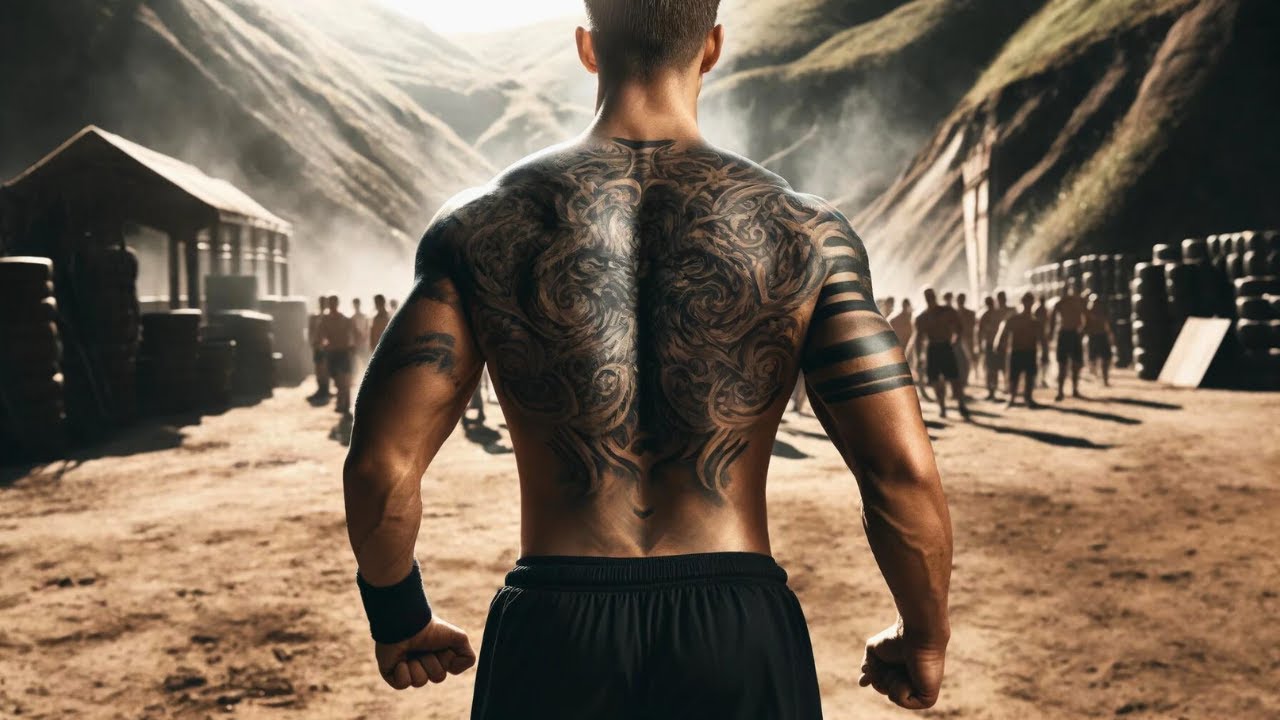A computer-animated or AI-generated image depicts a muscular, heavily tattooed man who appears to be in his 40s, standing shirtless in a fighting stance on a deck or driveway in front of a building. He has a grayish bushy beard and head of dark, partially graying hair. His skin is very tan, and he is extensively tattooed, including a prominent chest tattoo of a winged creature with the word "Knox" in the center, additional words and designs below the chest tattoo, a large tattoo on his stomach, and a sleeve on his right forearm. The man is covered in blood, with a bloody nose and visible cuts on his arms and shoulders. In his right hand, he holds a weapon resembling a knife with a metallic, possibly golden blade. The setting behind him includes a darkened or apocalyptic sky, a blurred vehicle, and a railing, adding to the sense of dramatic tension in the scene. He is wearing dark pants or blue jeans.